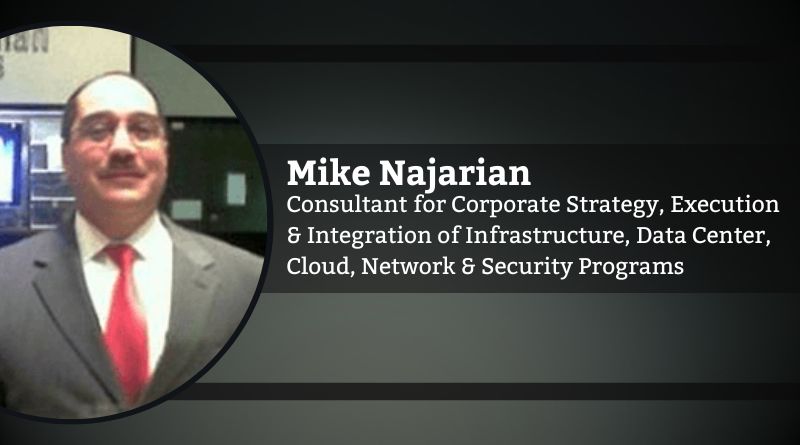This image features an ID bio card for Mike Najarian, a consultant specializing in corporate strategy execution and the integration of infrastructure, data center, cloud, network, and security programs. The card has a dark gray background with black stripes, transitioning into a softer gradient from black in the top right corner to lighter gray in the bottom left. Centered on the card, a bold black ribbon with white text displays Mike Najarian's name and professional title. A circular, albeit pixelated, photo of Mike is positioned adjacent to the text. In the low-quality image, Mike is smiling warmly at the camera, wearing glasses, a dark gray suit jacket, a white button-up shirt, and a red tie. He has a small mustache, very short, receding hair, and rosy cheeks. In the background of his photo, there are computer screens and a wall that transitions from gray to white or off-white, bordered in black.